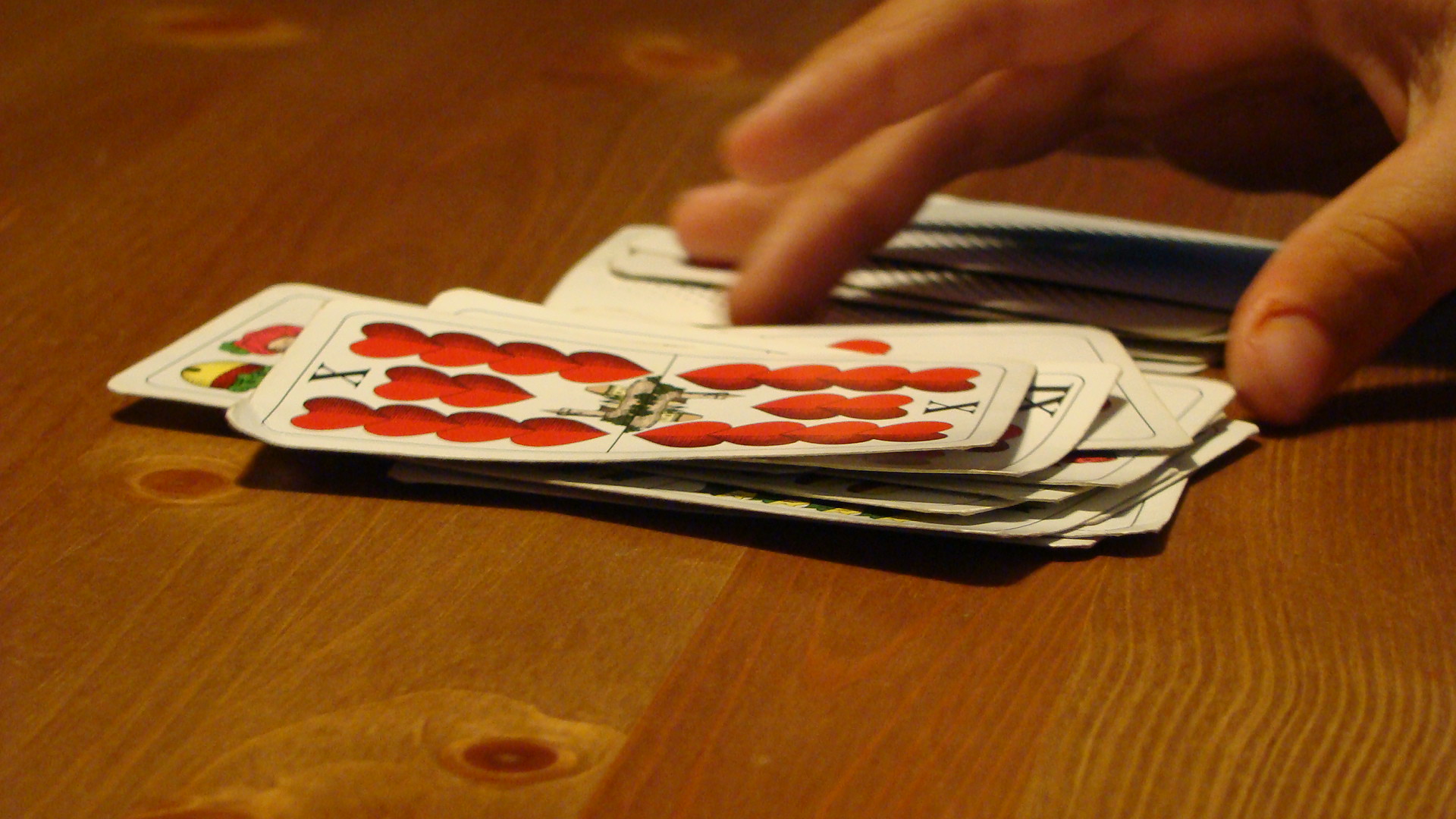A vibrant, landscape-oriented photograph captures a disordered pile of playing cards resting on a textured wooden surface, its grains and knots clearly visible. From the upper right corner, a partially cropped hand intrudes, its thumb and first three fingers extended toward the cards. Dominating the haphazard stack is the 10 of Hearts, distinguished by Roman numerals "X" at each end. The card features ten red hearts arranged in two rows of four with two in the center, flanking an indistinct illustration that appears to depict a castle or similar structure. The casual arrangement and tactile detail of the scene evoke a sense of impromptu play.